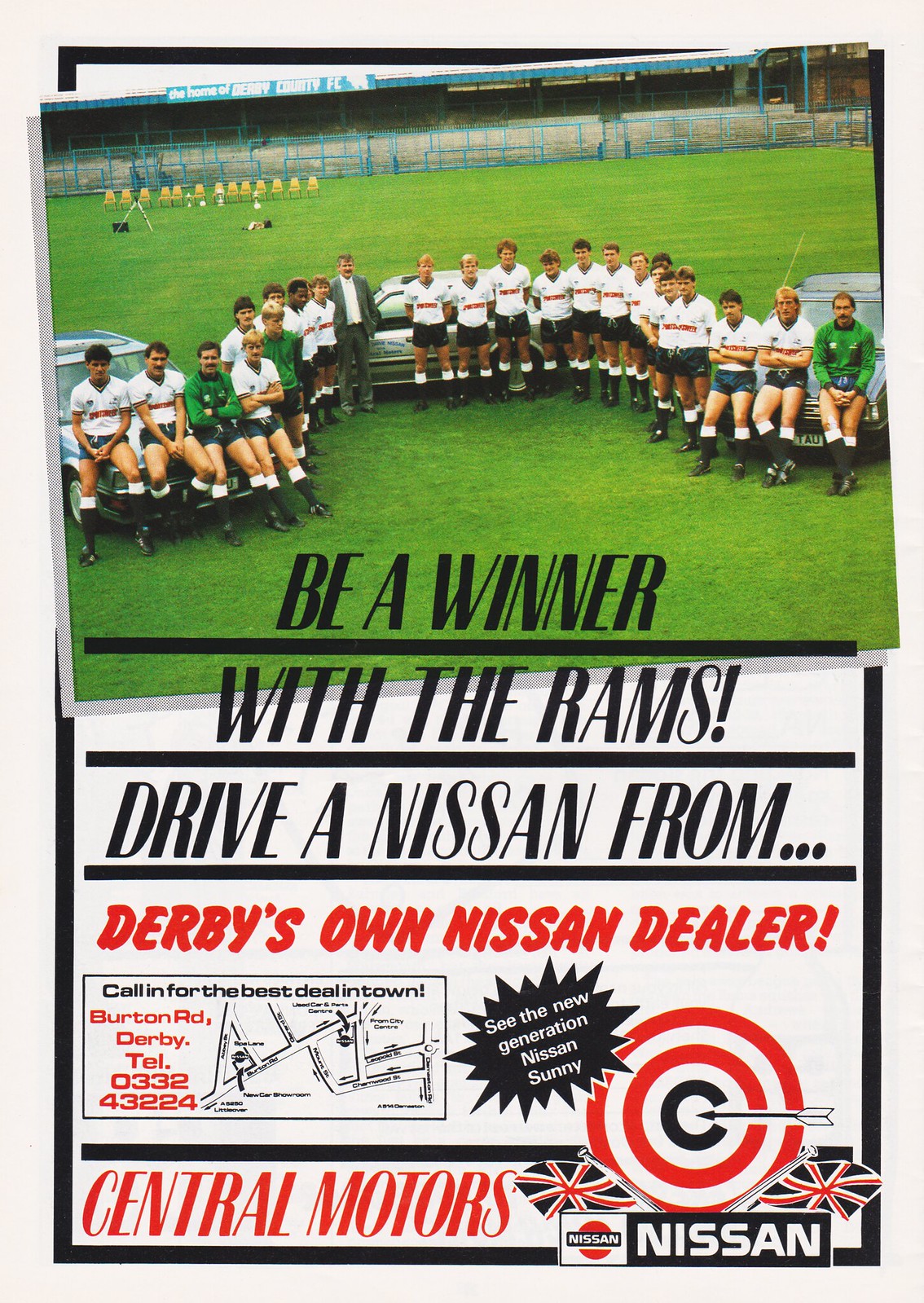This image appears to be a vintage full-page advertisement from a magazine, divided into an upper and lower section. The top half features a nostalgic photograph of a British soccer team, known as the Rams, posing on a lush green soccer field. The players, dressed in a mix of white jerseys and green shirts with dark navy blue shorts, are leaning against and sitting on three mid-70s to 80s Nissan vehicles arranged in a semicircular pattern. The background reveals empty stands, suggesting the photo was taken in an off-season or for promotional purposes.

Running across the bottom of the photograph and continuing into the lower half of the page is an advertisement with bold black text: "Be a winner with the Rams! Drive a Nissan from Derby's own Nissan dealer." Below this, in red lettering, it reads "Central Motors." The ad includes the Nissan logo, a small map with an arrow pointing to a target location, British flags, and further details encouraging readers to "see the new generation Nissan Sunny" and to "call in for the best deal in town." Contact information is provided, listing the address as Burton Road, Derby, and a telephone number, 0332-43224. This combination of imagery and text clearly positions the ad as a compelling promotion from Central Motors, aimed at enticing soccer fans to purchase a Nissan.